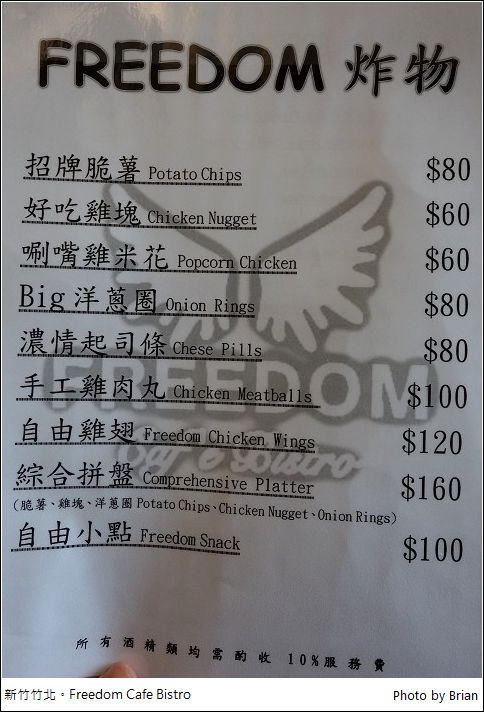The image depicts a menu from an establishment named the "Freedom Cafe and Bistro." The menu is held at the bottom by a thumb, with text primarily in English accompanied by what appears to be Chinese characters. The background of the menu is a slightly cream color, featuring a faded logo in the center that reads "Freedom Cafe and Bistro." Here are the detailed menu items listed, along with their respective prices:

1. Potato Chips - $80
2. Chicken Nuggets - $60
3. Popcorn Chicken - $60
4. Onion Rings - $80
5. Cheese Pills - $80
6. Chicken Meatballs - $100
7. Freedom Chicken Wings - $120
8. Comprehensive Platter (includes Potato Chips, Chicken Nuggets, and Onion Rings) - $160
9. Freedom Snack - $100

At the very bottom, additional text in Chinese characters indicates a 10% charge, possibly a service charge or discount. The right side of the menu notes that the photo was taken by someone named Brian.